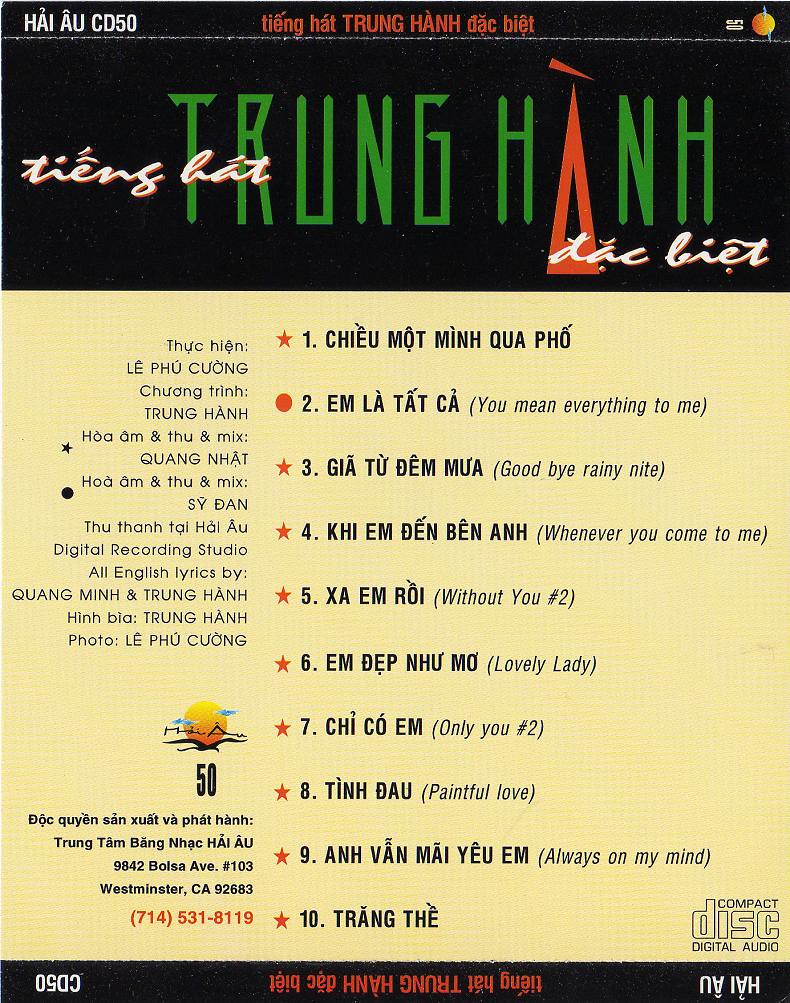The image depicts the cover of what appears to be a CD insert from an Asian, potentially Vietnamese, artist. The color scheme is predominantly black at the top with green text, and yellow at the bottom. At the top center of the cover, large green lettering spells "Trung Hành," with the 'A' stylized as a red triangle. Below the artist name, there is more text in a foreign language in white and red fonts. To the left bottom, a red phone number is visible. The phrase "CD 50" is present at both the top and bottom of the image. A compact disc digital audio logo is located at the very bottom right in black font, with "disc" highlighted in yellow. The bottom of the cover features a pale yellow background with blue text listing the songs. Tracks numbered 1 and 10 are purely in a foreign language, while tracks 2 through 9 include English titles such as "You Mean Everything to Me," "Goodbye Rainy Night," and "Always On My Mind." Additionally, there is a small image of an orange and yellow sun with clouds and a bird silhouette, placed near the bottom center of the cover with the number 50 inside it. Overall, the insert is text-heavy and largely incomprehensible without knowledge of the foreign language it is written in.